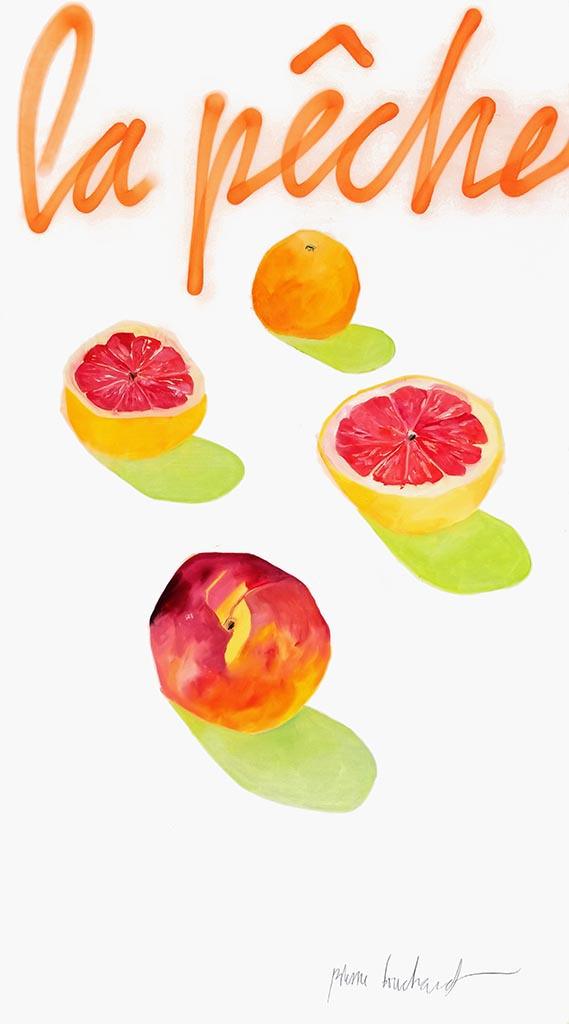This is an image of a watercolor painting titled "La Pêche," written in orange lettering at the top. The painting prominently features a variety of fruits. In the center, there are two halves of a grapefruit, depicted with yellow peels and vivid red interiors. Between the grapefruit halves lies a whole orange with a green shadow on its right side, a small black dot at the top indicating where the stem was. The fruits are all rendered with a green shadow, adding depth to the composition. The artwork is signed by the artist at the bottom, though the signature is not entirely legible, possibly reading "Pierre Bouchard." The painting rests on a plain white background, emphasizing the colorful fruits.